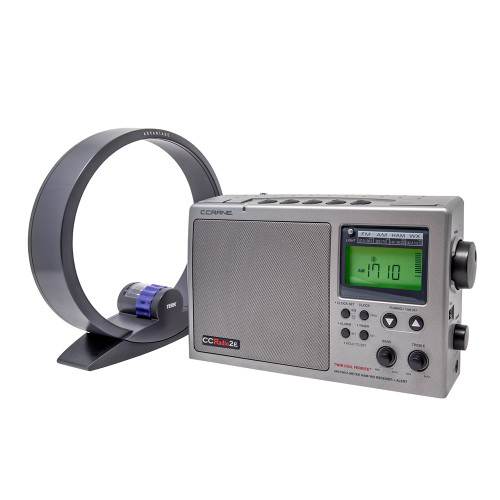The image displays a CC Radio 2, prominently set against a plain white background. This sleek, rectangular radio features a large gray speaker on the front, with the brand name "C. Crane" embossed at the top. The model label "CC Radio 2" is also visible. Five circular buttons with embossed symbols for play, pause, and stop are aligned across the top of the radio. On the right side, there are two black dials, with the larger one being about the size of a dime, and a headphone jack situated at the bottom right. The front of the radio also showcases a green digital display reading "1710" for the tuning station. Below this display are various buttons and dials for tuning, bass, and treble adjustments. To the left of the radio stands a curved, dark gray antenna with a distinctive circular design, featuring a small trapezoidal base and a blue bumpy dial at the bottom. The object appears to be slightly angled towards the center-left of the image, enhancing its three-dimensional appearance.